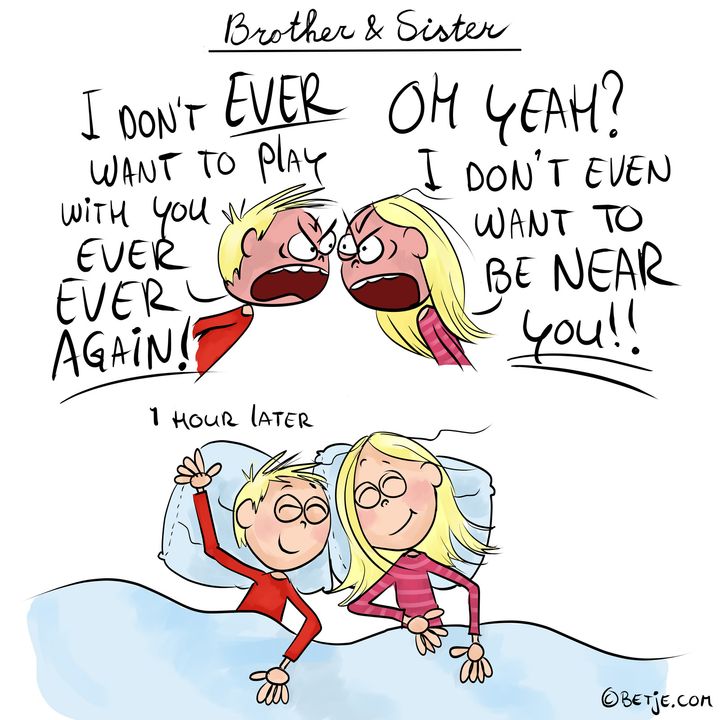The colorful illustration, titled "Brother and Sister," shows two blonde-haired siblings at the center of a playful comic-style poster. In the top part of the image, the brother, wearing a red shirt, stands on the left, angrily yelling, "I don't ever want to play with you ever again," while the sister, in a light pink and dark pink striped shirt on the right, retorts, "Oh yeah, I don't even want to be near you!" Both children have furious expressions, with red faces signaling their anger. Above them, a script in black that reads "Brother and Sister" is underlined.

Below this scene, another illustration shows the siblings an hour later, happily reconciled. Lying in bed with blue pillows and a blue blanket, they are smiling with their eyes closed, clearly content and at peace. The text "one hour later" appears in black above the boy's head on the left, capturing the swift change from conflict to harmony. At the very bottom right of the image is a small trademark symbol and the text Bet J E dot com. This charming depiction highlights the fleeting nature of sibling spats and their enduring bond.